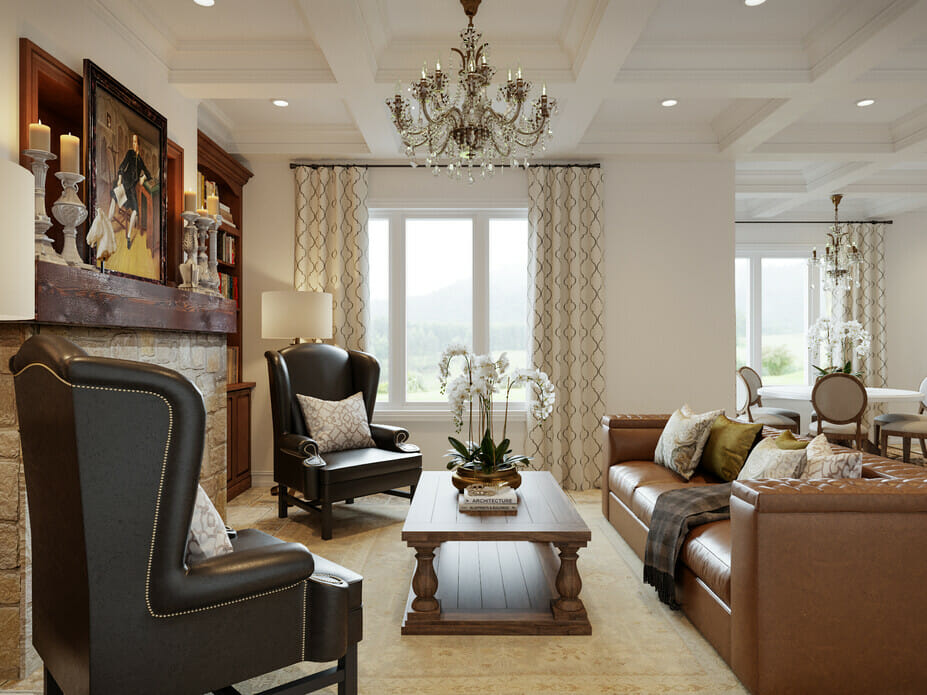This image showcases a sophisticated, rustic-modern living room that transitions into a dining area. The formal living room features understated beige walls and a ceiling adorned with white beams and a resplendent chandelier, detailed with diamond-like clear elements and white lights atop a silver frame. A prominent stone fireplace, crowned with a dark brown wooden mantel, anchors the room. The mantel is decorated with off-white candles and a portrait of a distinguished gentleman in a black cloak, holding a white paper, framed by black and brown wood. A white horse head statue adds a unique charm to the mantelpiece. Flanking the fireplace are two black leather wing chairs with throw pillows, creating a cozy reading nook.

Centering the room is a dark wooden coffee table, supported by ornate spindles, and topped with a white floral centerpiece. To the right, a plush tan leather couch is adorned with gold, white, and brown pillows, complemented by a dark throw blanket. Behind this setup, elegant white curtains with darker tan and black designs frame large windows, providing a serene view of a mountain environment.

An adjacent dining area can be seen behind the sitting room, distinguished by a white dining table surrounded by matching chairs, all accented with gold trim. The dining space is illuminated by a gold and diamond-like chandelier. The flooring throughout both rooms consists of warm brown wood, and a white, gold, and gray rug underlines the coffee table in the living room. Lastly, a brown wooden bookshelf filled with a variety of books stands near the windows, adding to the room's intellectual atmosphere.